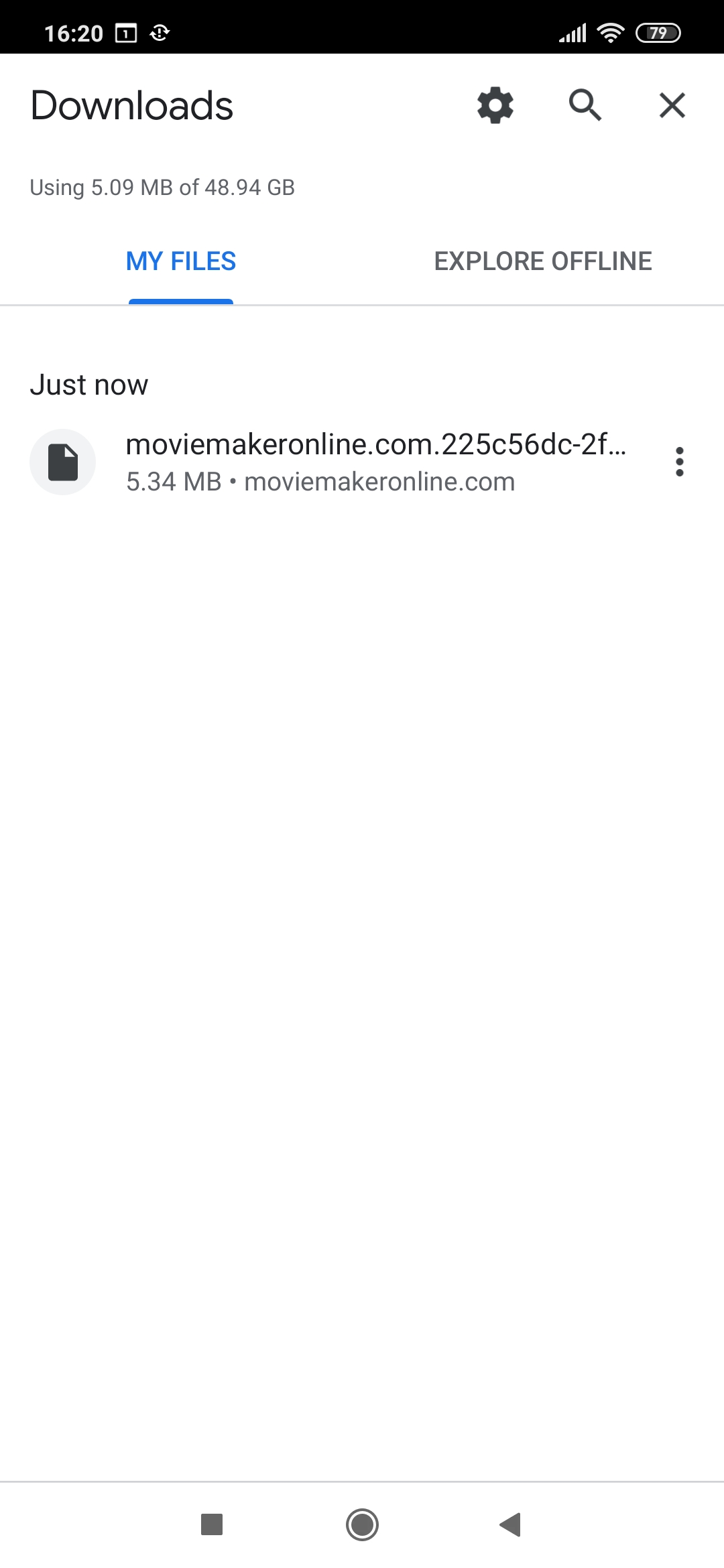Displayed in the image is a digital interface showcasing download progress and various system settings. The download bar indicates that 5.09 megabytes have been downloaded out of a total capacity of 48.94 gigabytes. Icons and labels are arranged to represent different functions: a file exploring option for offline use, a Movie.com maker utilizing 5.34 megabytes, and geometric icons including a square, circle, and triangle. Additionally, there are settings and search functions, denoted by an 'X' symbol. In the top right corner, the screen displays Wi-Fi connectivity at 79% and battery life status. A calendar marked as 1620 is circled, and a cluster of four lines suggests a menu or list option. At the bottom, a "Thanks for watching" message concludes the display.